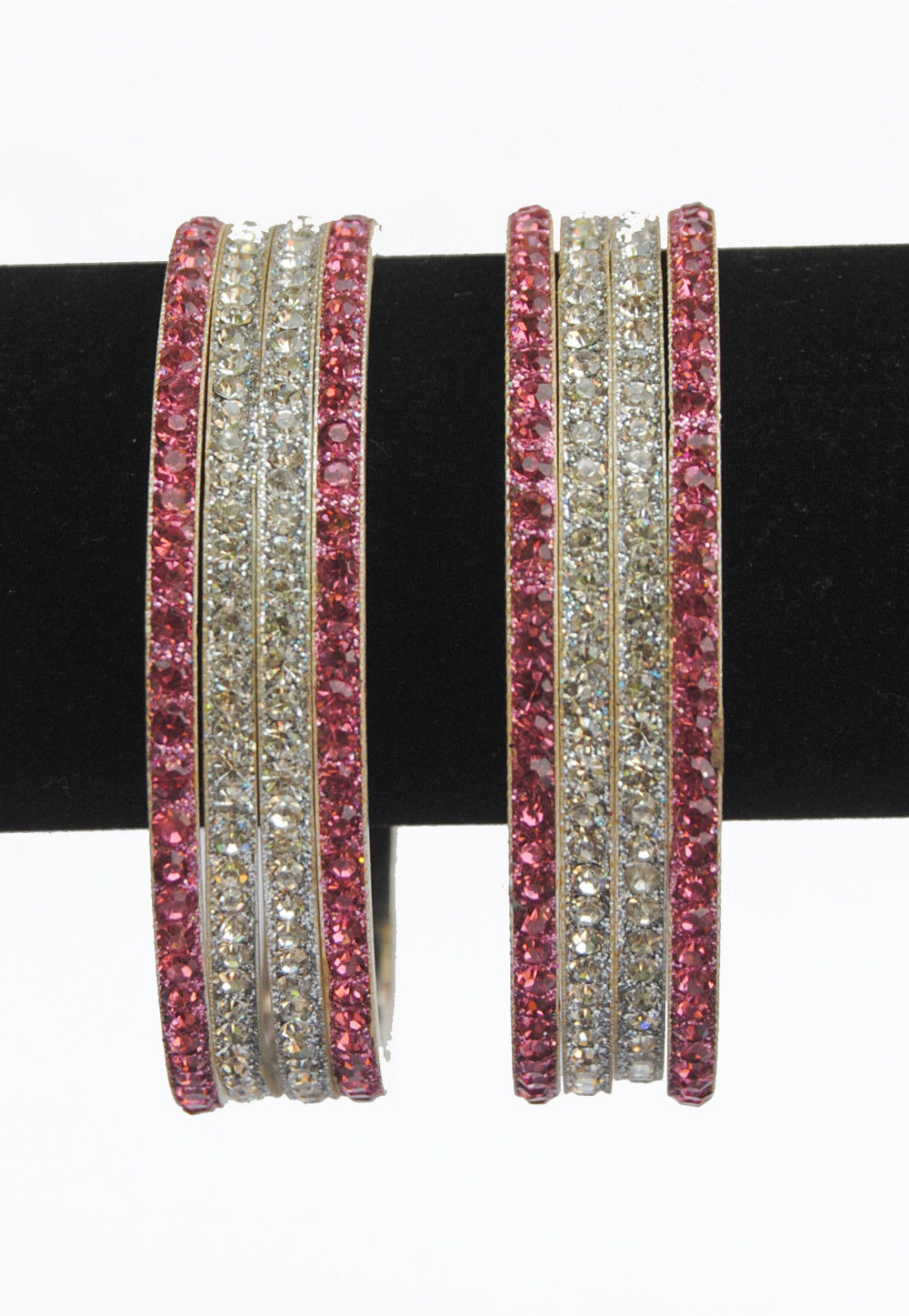Displayed against a black tubular stand, zoomed in to show only a section, appears to be a pair of identical bracelets. The stand itself is cropped, leaving the bracelets as the main focal point. Each bracelet features four rows of gemstones arranged in a distinctive pattern. The outermost rows are adorned with vibrant pink gemstones, while the two center rows glisten with clear, diamond-like stones. The partial view of the bracelet on the left reveals a hint of a silver edge, suggesting the bracelets are set in silver. The intricate design and the reflective quality of the stones make this display both elegant and eye-catching.